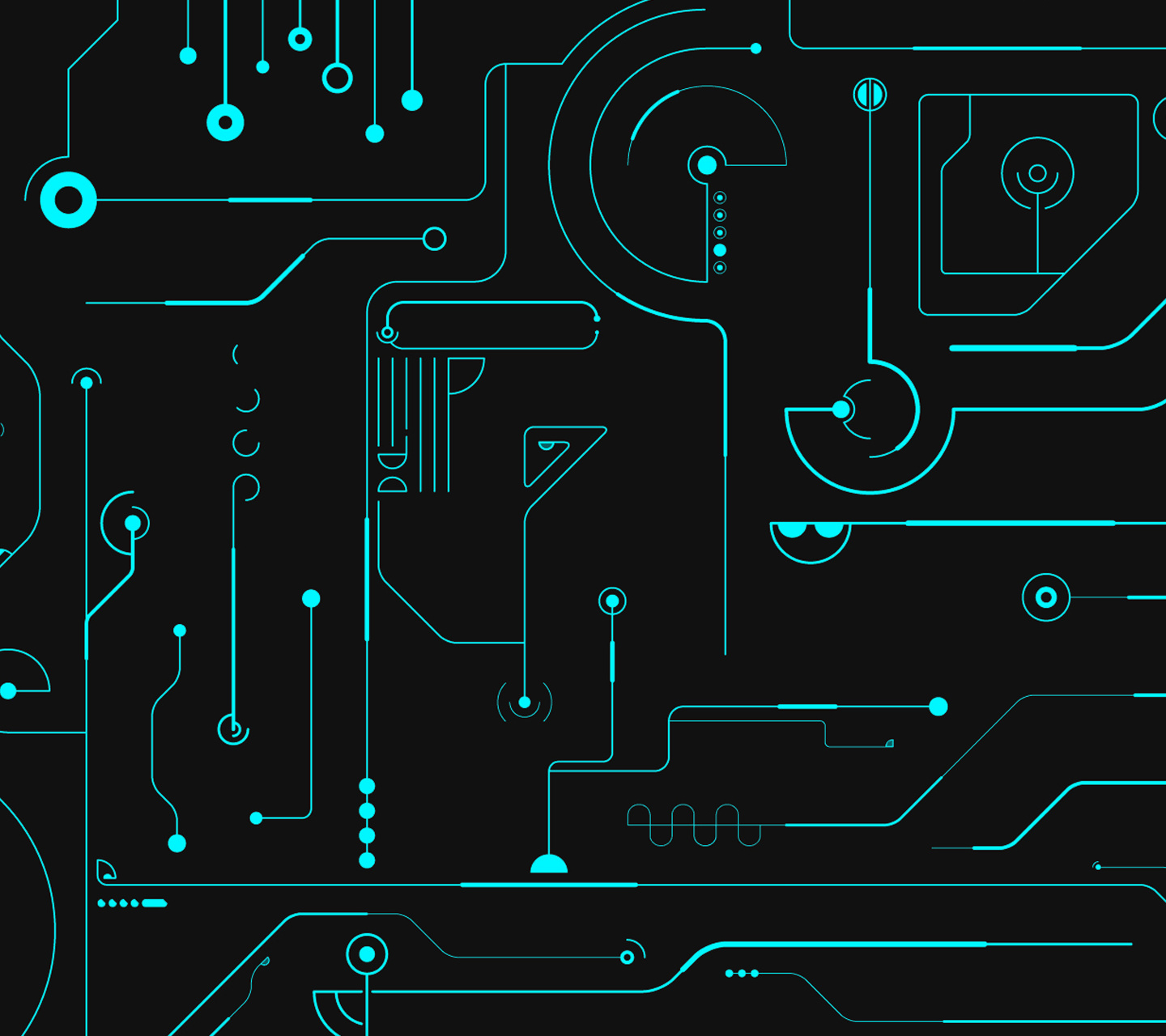The image is a futuristic drawing set against a completely black background. The drawing is composed entirely of aqua green or light blue elements, consisting of numerous lines, circles, and various designs. These lines vary in thickness and length, with some being straight and arranged both horizontally and vertically, while others are curved. In the upper left corner, several circles with black centers dangle from thin lines, resembling strings. To the right, there is another prominent outlined circle. The intricate network of lines and shapes is reminiscent of the complex wiring found on a motherboard, yet it doesn't form any discernible pattern or spell out anything specific. Despite the chaotic appearance of lines and circles, the overall effect is striking and visually intriguing, evoking the feel of neon lights.